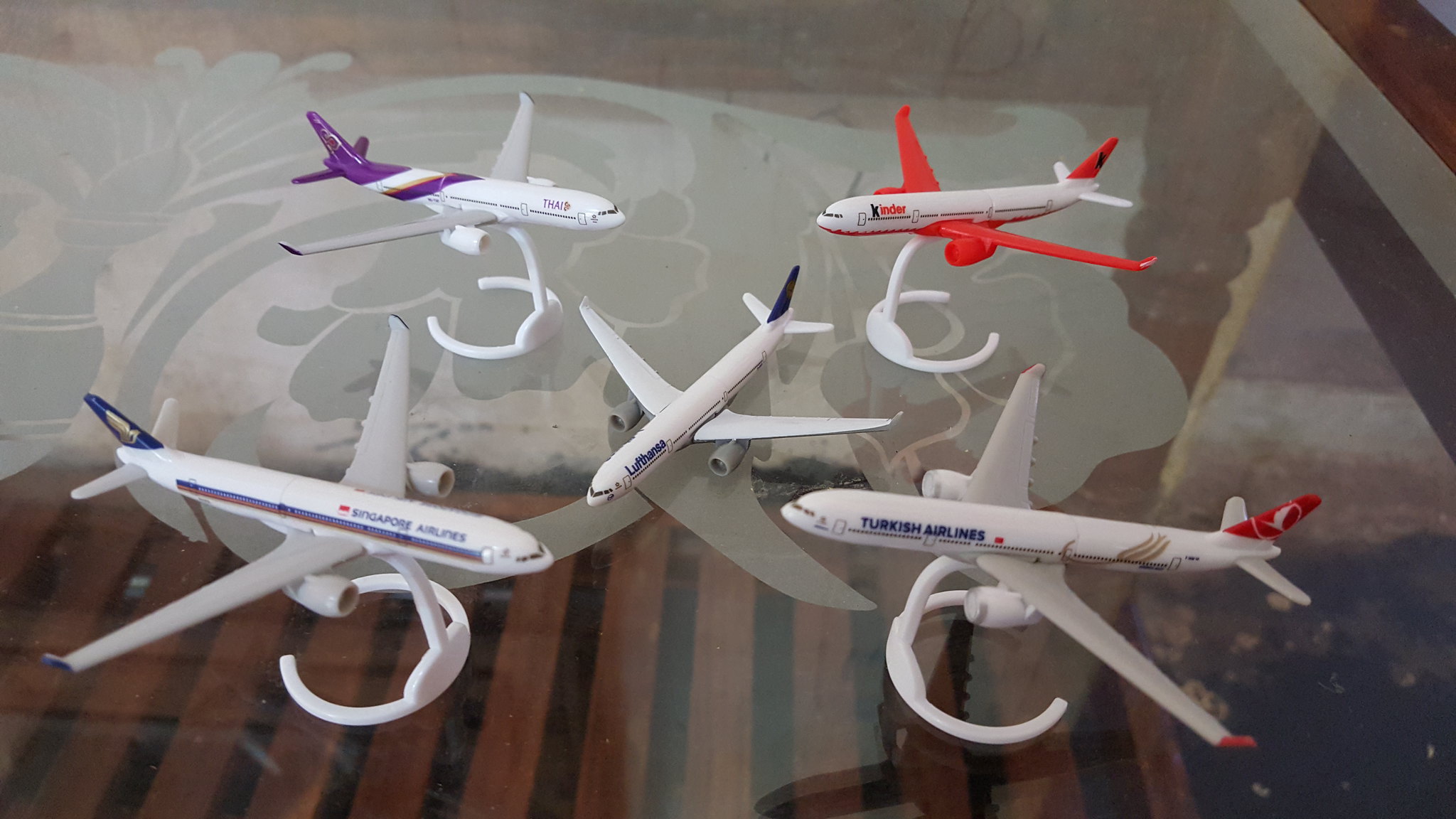This color photograph captures five model airplanes displayed on a reflective glass coffee table, which features a smoky floral decal in the center. The table, with a dark wooden border and legs, has a shelf of brown wooden slats visible beneath the glass surface. Each plane is perched on a white stand, creating the illusion of flight. The arrangement consists of four planes facing towards the center and one in the middle facing the viewer, adding symmetry and balance to the display.

Starting from the upper left, the first airplane showcases a purple tail with yellow and purple stripes. The upper right plane has distinctive red wings and tail. The lower left airplane features a navy blue tail, while the lower right one sports a red tail and blue "Turkish Airlines" lettering with gold accents. The central airplane has a navy blue tail and faces outward towards the photographer. The combination of the table’s reflective properties and the careful arrangement of the model airplanes emphasizes their details and colors, while the floral etching in the glass adds a delicate touch to the overall composition.